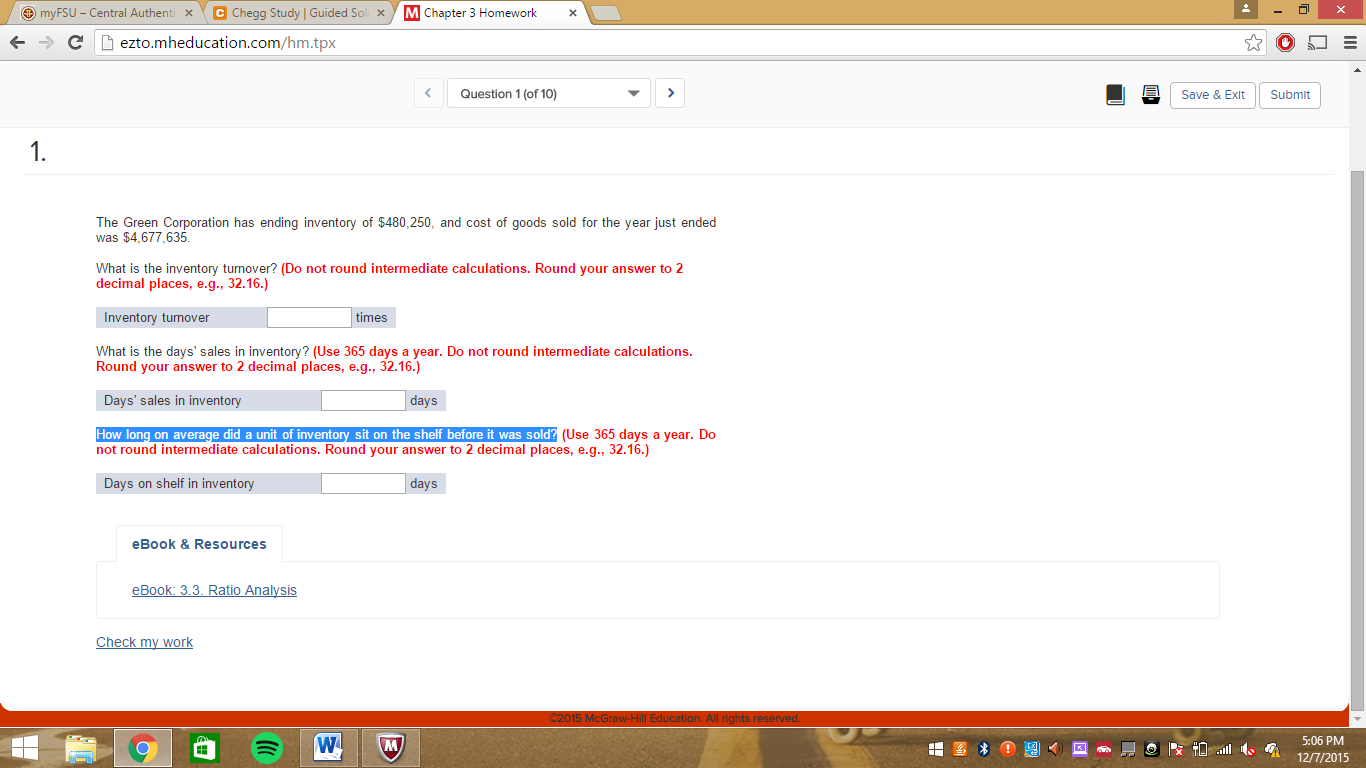The screenshot displays an online classroom interface. The browser has three tabs open. The first tab, not highlighted, is labeled "My FSU Central Authentication." The second tab, also not highlighted, is partially titled "Chegg Study Guided," but the rest of the text is obscured. The currently active third tab is labeled "Chapter 3 Homework," with the URL displayed as "ezto.mheducation.com/hm.tpx."

At the top of the screen, a navigation bar indicates "Question 1 of 10." Below this, the main content area presents a homework question with detailed descriptions and instructions highlighted in red. The interface includes several input fields for entering responses, specifically numbers or days related to the question.

Further down, a section titled "eBook and Resources" offers two links: "eBook 3.3 Ratio Analysis" and another link labeled "Check My Work" for verifying answers. At the bottom of the screen, a small red-bordered area contains copyright information.

The desktop taskbar at the very bottom shows icons for Google Chrome, Microsoft Word, and a third icon, gray with a red center, resembling the logo of Adobe Acrobat or a similar application with an "M" in the center.